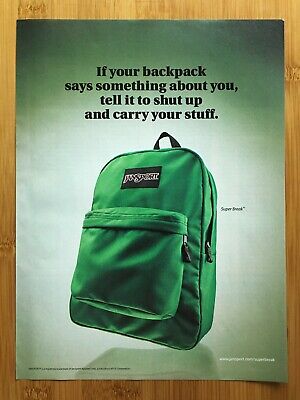The advertisement poster, prominently placed on a light brown wooden surface, features a humorous and striking design. The rectangular poster has a soft gradient background, transitioning from a lighter white in the center to vibrant green hues around the edges, culminating in black at the top corners. At the top center of the poster, bold black text reads: "If your backpack says something about you, tell it to shut up and carry your stuff."

Beneath this catchy slogan, a photograph of a vibrant green Jansport backpack is prominently displayed. The backpack is angled slightly to the left, showcasing its black top strap and a small black label with dark maroon lettering, too fine to be legible. This green backpack is detailed with a second compartment featuring a zipper on the right side with a black handle. Additionally, there are three smaller texts in black and white spotted in the bottom corners and next to the backpack, though their resolution is too low to discern their contents. The entire advertisement exudes a mix of practicality and humor, vividly capturing attention against the wooden backdrop.